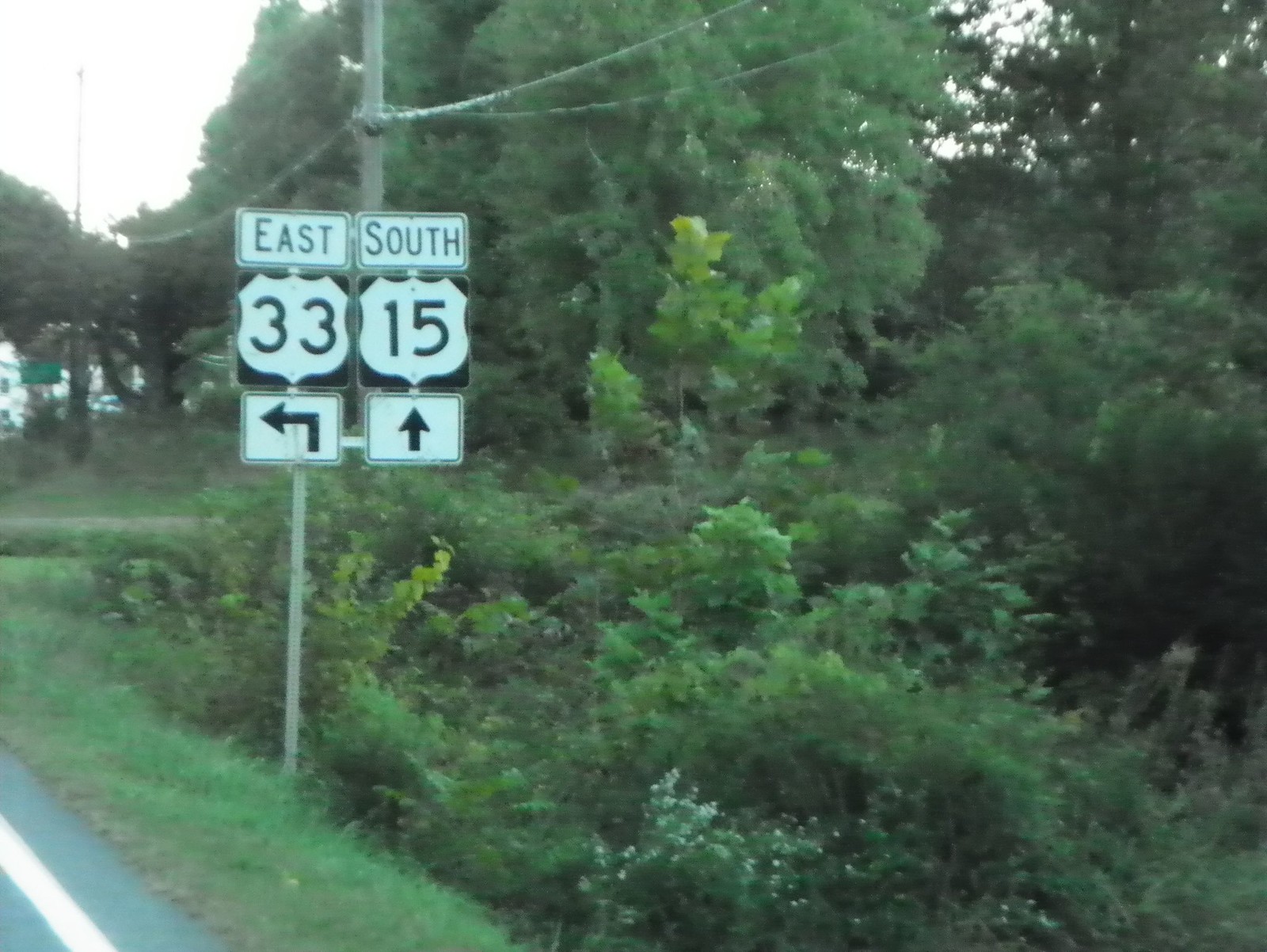The image captures a wooded roadside scene with a glimpse of the road's lower left corner, marked by a white border stripe. Prominent in the foreground are two state route signs affixed to a pole. The left sign indicates Route 33 East with a left turn arrow below it, while the right sign denotes Route 15 South with a straight-ahead arrow. Surrounding the signs, the area transitions from grass to shrubbery and then to tall trees, suggesting a dense and untamed environment. Telephone wires run parallel to the road, supported by power poles, one of which is visible near the signs. A small intersecting road is partially visible on the left side, with a green sign in the distant background and possibly a fallen tree just behind the road signs.